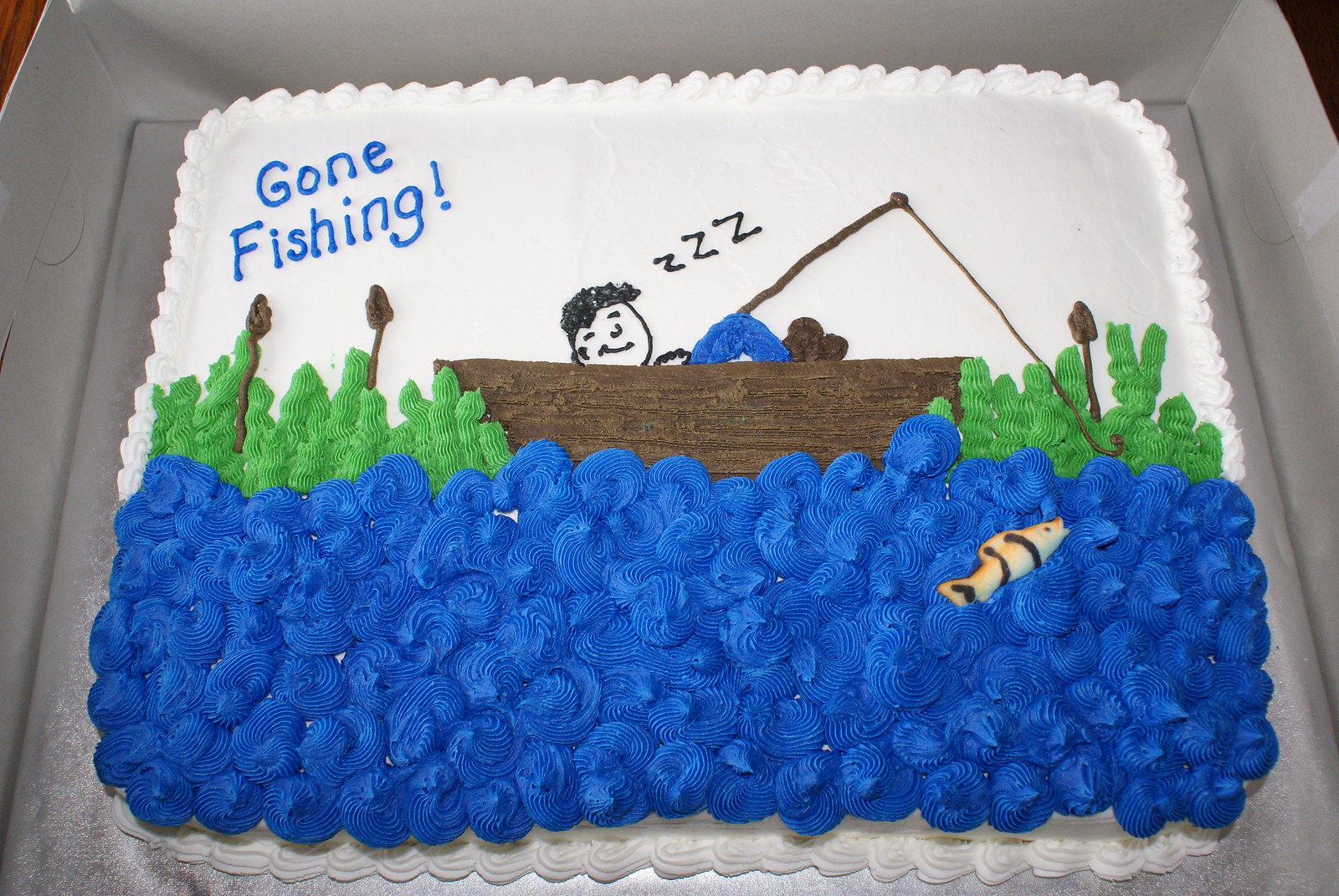In this detailed and colorful photograph, we see a cake placed inside a white box on a possibly wooden surface, suggesting an indoor setting like a kitchen or a bakery. The cake itself is a rectangular, landscape-oriented masterpiece, featuring intricate icing decorations. 

The upper portion of the cake has a white background mimicking the sky, with the top left corner displaying the words "Gone Fishing" in blue icing. Below this, a green horizon line dotted with trees spans the width of the cake, setting the scene. 

The central focal point is a brown boat, where a stick figure man is seen reclining, smiling, and holding a fishing pole. Above his head, the letters "ZZZ" indicate that he is sleeping. Plants and cattails, crafted from green and brown icing, surround the boat, adding to the natural ambiance. The bottom half of the cake features blue icing with swirls representing water; a gold fish is depicted approaching the man’s hook in the right corner. The cake rests on a white tray, combining elements of photographic realism with representational artistry.